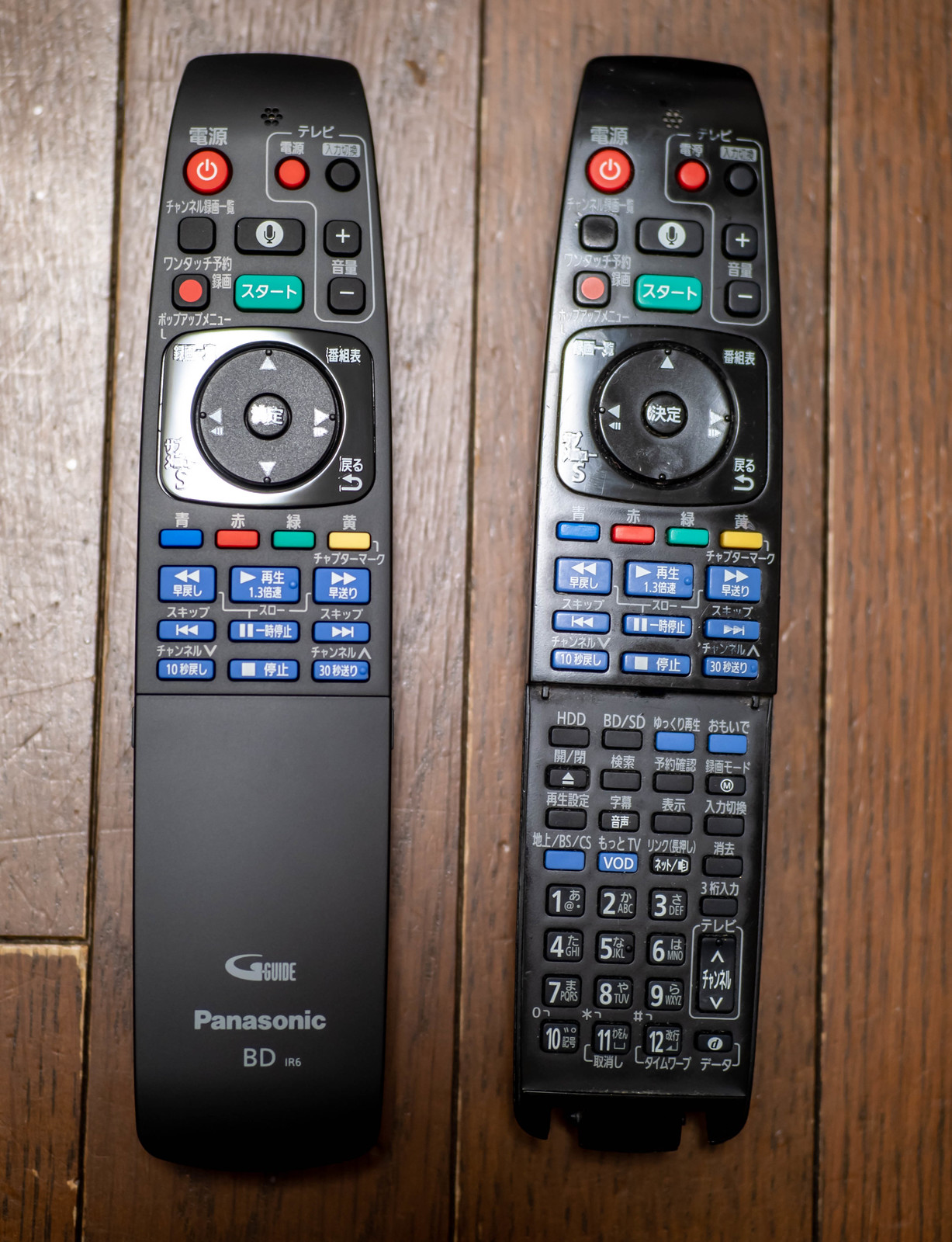This image features two long, narrow remote controls placed parallel to each other on a dark brown wood plank surface, likely a wooden table or floor. Both remotes are predominantly black and feature Asian characters, indicating they are designed for an Asian market. The remote on the left includes a distinct red power button at the top, a circular button with directional arrows in the center, followed by four buttons below it and additional blue buttons further down labeled for functions like Panasonic BD Guide. The remote on the right, similar in size and appearance, also features buttons below the blue keys, including numbers and additional black and white keys. Both remotes display a mix of various colored buttons, including red, blue, black, yellow, and green, and their function labels are all in Chinese or Japanese characters.